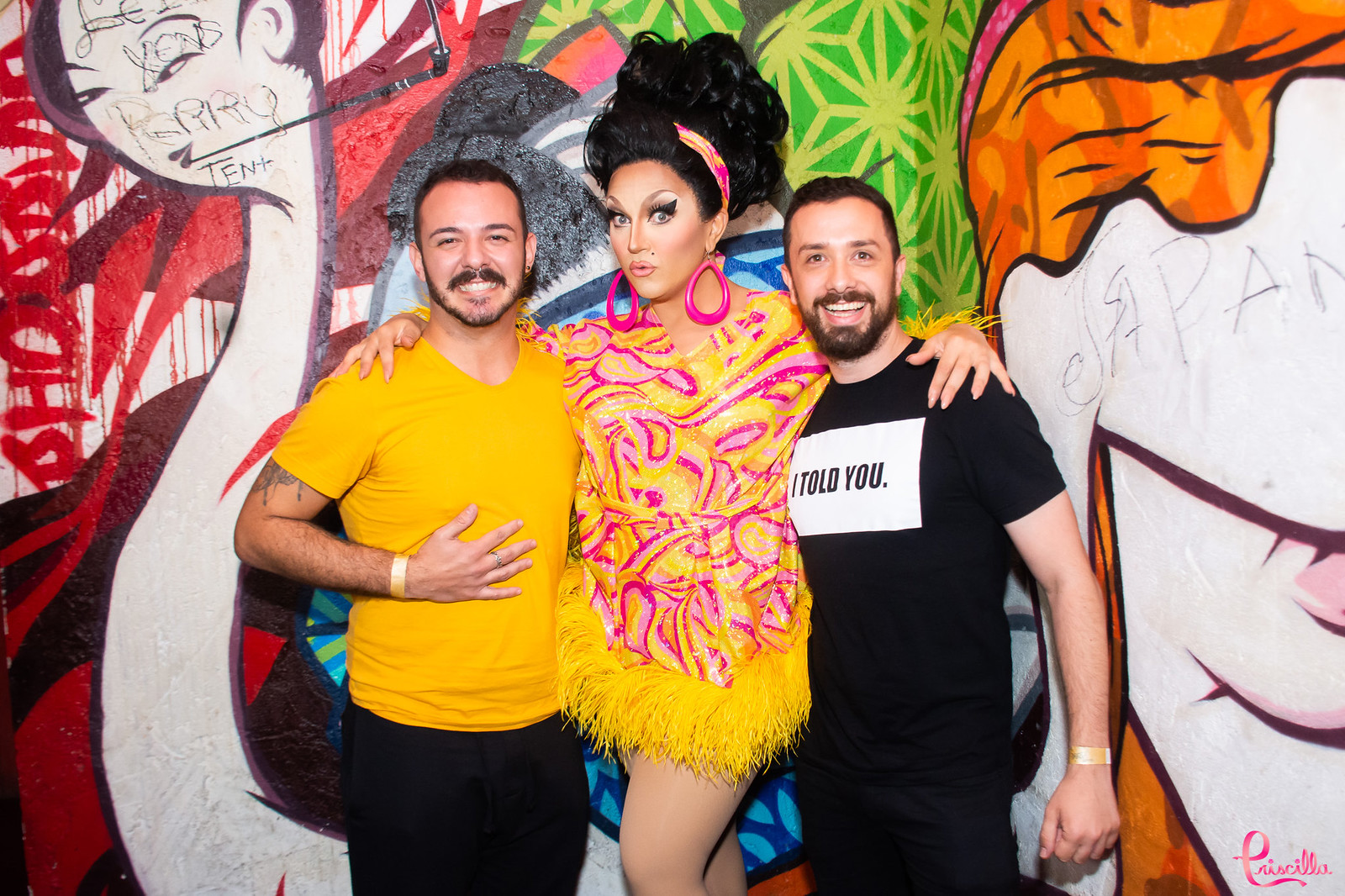This captivating photograph showcases three striking individuals standing together in front of a vibrant, graffiti-style mural, likely taken outdoors. In the center of the group, a charismatic drag queen dominates the scene with her bold, colorful ensemble reminiscent of 70s fashion. She is adorned in a head-turning fringed dress featuring hues of yellow and pink that perfectly match her large pink hoop earrings and her elaborate yellow and pink headband. Her dramatic eye makeup, including heavy eyeliner, and her voluminous, dark updo complete her glamorous look. 

On either side of her stand two men with beards and mustaches. The man on the left is dressed in a yellow short-sleeve t-shirt, revealing a tattoo above his elbow and a yellow bracelet on his wrist. His arm, bent at the elbow, rests casually against his torso, where he also wears a ring on his middle finger. The man on the right sports a black t-shirt emblazoned with the white text "I told you." He also has a paper wristband on, suggesting this photo was taken at an event.

The background mural is a riot of colors—red, white, green, black, orange, and blue—featuring imaginative, abstract representations of faces. One face, distinctly of an Asian woman with "Japan" scribbled over it, has a long neck reminiscent of a flamingo, while another figure seems to have long orange hair, an open mouth, but no eyes. Additional graffiti-like scribblings can be seen, adding to the mural’s chaotic yet artistic vibe. In the bottom right corner, elegant pink cursive text spells out "Priscilla," possibly hinting at the event or the artist's name. The mural's vibrant and eclectic elements serve as a compelling backdrop, perfectly complementing the vivid and lively attire of the central figure.